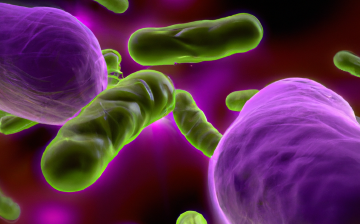The image is a highly magnified digital rendering of cells, potentially representing bacteria or a virus within a biological environment such as an animal or human. The background features an out-of-focus, gradient of purples with a reddish tint, creating a deep, mysterious ambiance. Dominating the scene are numerous cylindrical, capsule-shaped green structures, reminiscent of elongated hot dogs, scattered throughout the image. Among these green entities, two larger, smooth purple masses with slightly dimpled surfaces can be seen, floating prominently. There are no labels provided, leaving the exact identification of the cells and their context ambiguous.